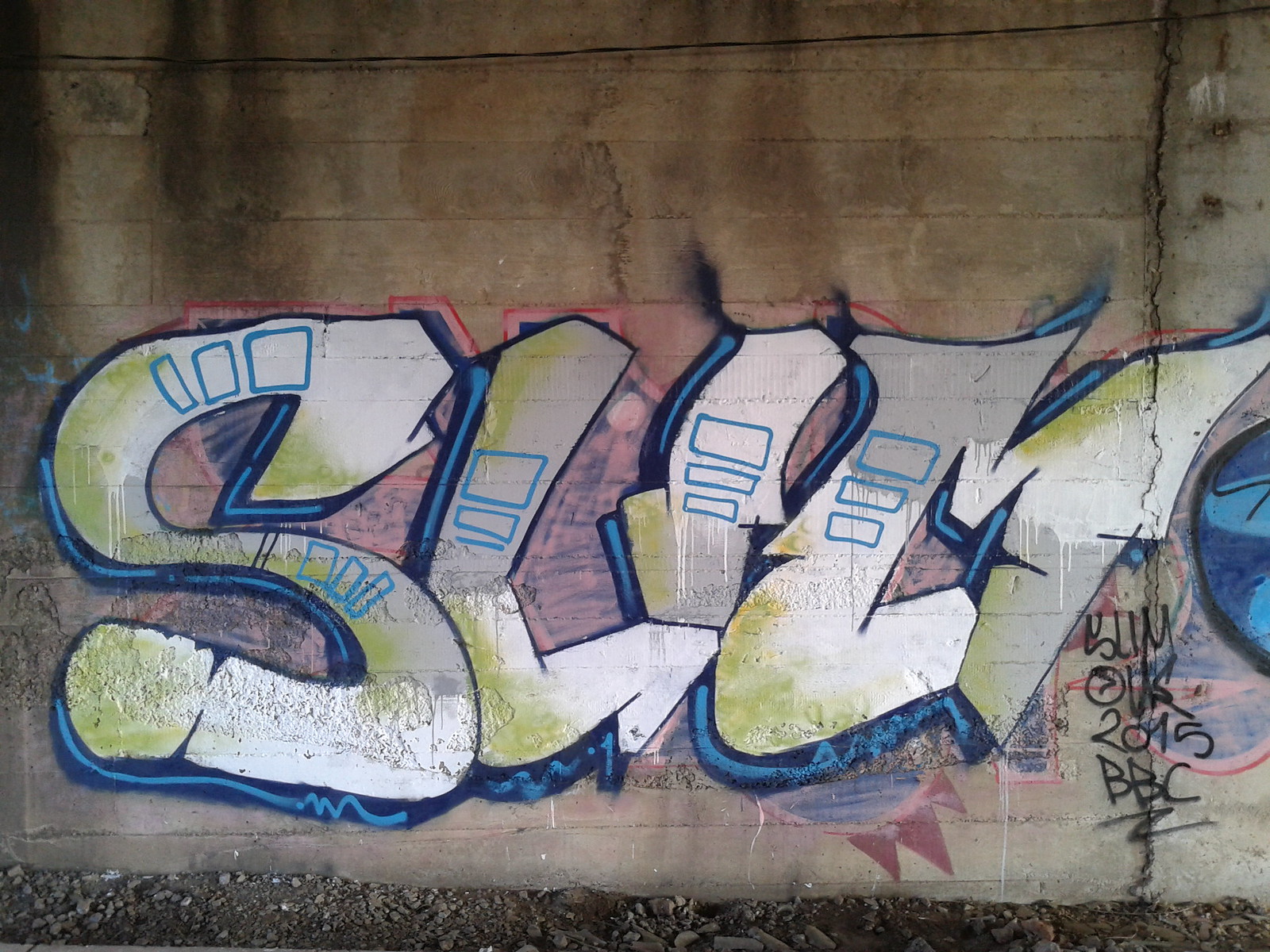The image depicts an old, cracking, concrete wall, possibly the underside of an overpass support or bridge, enveloped in dim, cloudy light. Dominating the wall is a prominent piece of graffiti featuring the word "Slim" rendered in typical graffiti style, with grays and whites accented by blue shadows. The letters incorporate blue squares and rectangles, adding depth and texture to the otherwise muted color palette. Below this large tag, in the bottom right corner, lies a smaller inscription reading "Slim OK 2015 BBC." The ground beneath the wall is strewn with gray rocks, emphasizing the aged and neglected state of the surroundings.